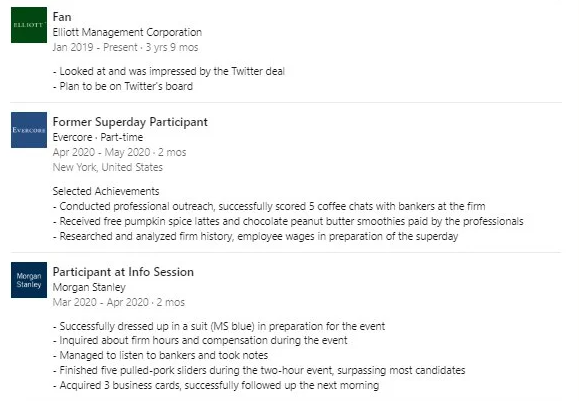Here is a detailed descriptive caption for the image:

---

The image showcases several significant messages and achievements of an individual, highlighting key experiences spanning over a few years. First, it references communications from FAN and Elios Management Corporation dated January 2019, indicating a three-year and nine-month period during which the individual observed and expressed admiration for a Twitter deal and planned to join Twitter's board. 

Subsequently, the image mentions the individual's involvement as a former Super Day participant in a part-time role from April 2020 to May 2020 in New York, United States. During this period, notable accomplishments include conducting professional outreach and successfully arranging five coffee meetings with bankers at FAN. As a gesture of networking, the individual received complimentary pumpkin spice lattes and chocolate peanut butter smoothies, courtesy of the professionals. Additionally, extensive research and analysis were conducted on FAN's history and employee wages in preparation for an Info Session dedicated to Super Day participants.

Furthermore, the image details the individual’s time at Morgan Stanley from March 2020 to April 2020, highlighting their successful attire in a suit, specifically MS Blue, as part of their professional preparation.

---